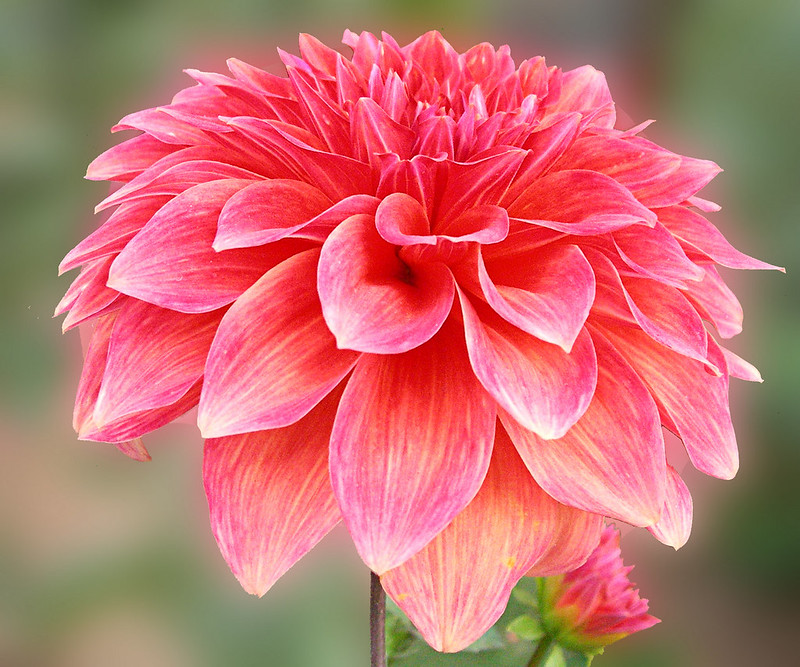The image is a close-up photograph capturing the exquisite details of a fully bloomed dahlia flower with a very shallow depth of field. The central focus is on a large, deep pink dahlia adorned with vibrant, colorful petals that feature subtle white tips and yellow striations. This richly hued flower is set against a blurred background, which enhances its sharp and vivid imagery. Directly behind and slightly to the lower right of the main flower, a smaller dahlia bud, still closed, can be seen, adding depth and a sense of progression to the composition. The stem of the central flower is partially visible and appears dark brown, providing a striking contrast to the brilliant petals. The overall setting suggests a garden with softly muted lighting that preserves the realistic color palette and natural beauty of the flowers.